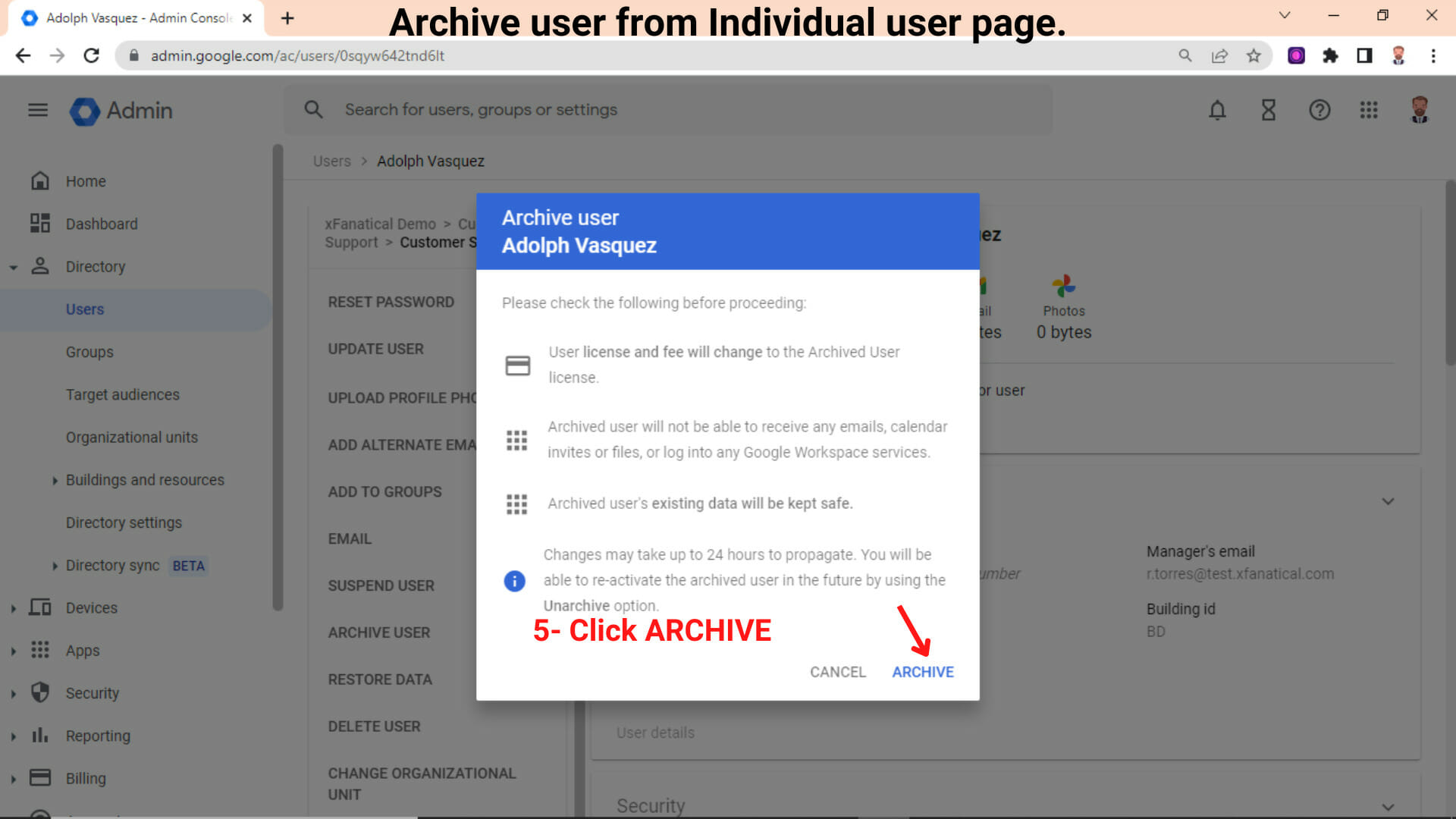The image features a detailed user interface pop-up related to archiving a user in a software application. The visual elements and text are as follows:

At the top, the background exhibits a peach color with a light gradient. A gray tab with a blue hexagon or octagon symbol is present. Inside the tab, in black text, it reads "Aldorf Asquest-Admin, CONSOL" alongside a black "X" and a black plus sign.

Beneath this tab, the bold, black text reads, "Archive User from Individual User Page". The underpinning background is gray due to an active pop-up.

The pop-up itself is predominantly a white rectangle with a blue header. At the top of the pop-up, white text declares, "Archive User Aldorf Asquest". Below, the pop-up displays an instruction: "Please check the filename before proceeding. User License and Fee would change to Archive User License. Archive User will not be able to receive any emails, calendar invites, or files, or log into any Google Workspace services. Archive User's existing data will be kept safe." 

To the left of an informational icon, a blue circle with a white 'i,' additional information is provided in small text: "Changes may take up to 24 hours to propagate. You'll be able to reactivate the Archive User in the future by using the Unarchive button."

At the bottom of the pop-up, a red label shows "5-Click Archive," followed by two buttons: "Cancel" in black and "Archive" in blue, with a red line pointing toward the "Archive" button.